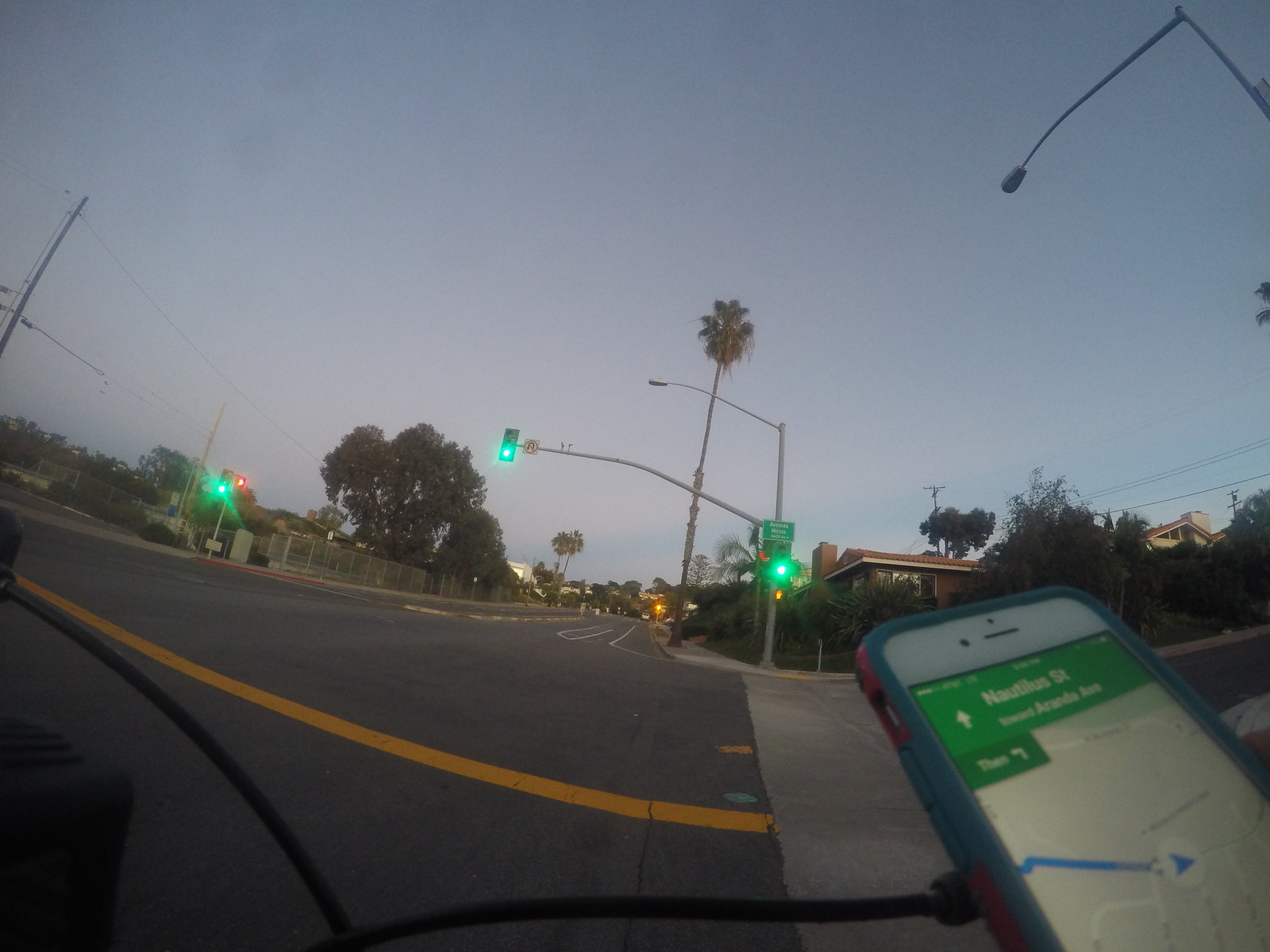A photograph captured from the windshield of a car offers a unique perspective, though it is slightly distorted with the sides of the street appearing to curl upwards. The scene features a black macadam road ahead, prominently marked by a bright yellow line. A green traffic light hangs at the intersection ahead, comprising three distinct green signals. Beyond the intersection, white lines are visible on the pavement. Notably, the road is devoid of any vehicles except for the car from which the photograph is presumably taken.

The backdrop is punctuated by a tall palm tree standing in the center, flanked by various deciduous trees on both sides. Inside the vehicle, an iPhone is visible on the dashboard, connected with a black cord. The iPhone, encased in blue, displays MapQuest with a blue directional arrow pointing towards an unreadable street name, likely beginning with an 'N' and featuring a green background.

The overall ambiance suggests dusk, as the sky transitions from a light blue to a dusky blue-gray, indicating the approaching sunset.